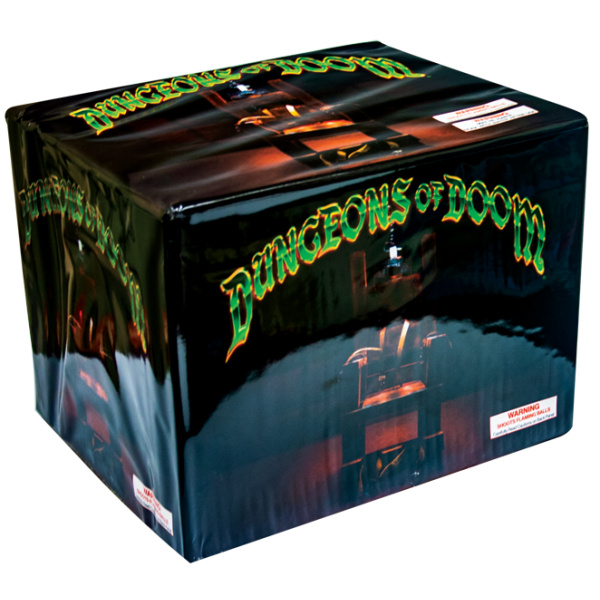The image depicts a three-dimensional box against a white background, primarily in black with three visible sides showcasing the title "Dungeons of Doom." The title, written in bold, all-caps green letters with a flame-like gradient from darker green at the top to lighter green at the bottom and outlined in shimmering gold, stands prominently on the front cover, top, and visible side of the box. Dominating the front cover is a detailed, dimly lit illustration of a brown wooden electric chair, complete with a silver cap hanging over it and leather straps intended for restraint, conveying a sense of impending danger. The same haunting image repeats on the top and side of the box. The box is wrapped in a slightly wrinkled plastic that reflects light, hinting at the packaging's texture. Prominent warning labels with red lettering on a white background are visible on every side, though the specific warning text is blurred, suggesting a potential hazard, possibly relating to flammability. This consistent artwork and text design suggests a cohesive, possibly ominous theme, potentially indicating a board game or a computer game themed around perilous adventures in the "Dungeons of Doom."